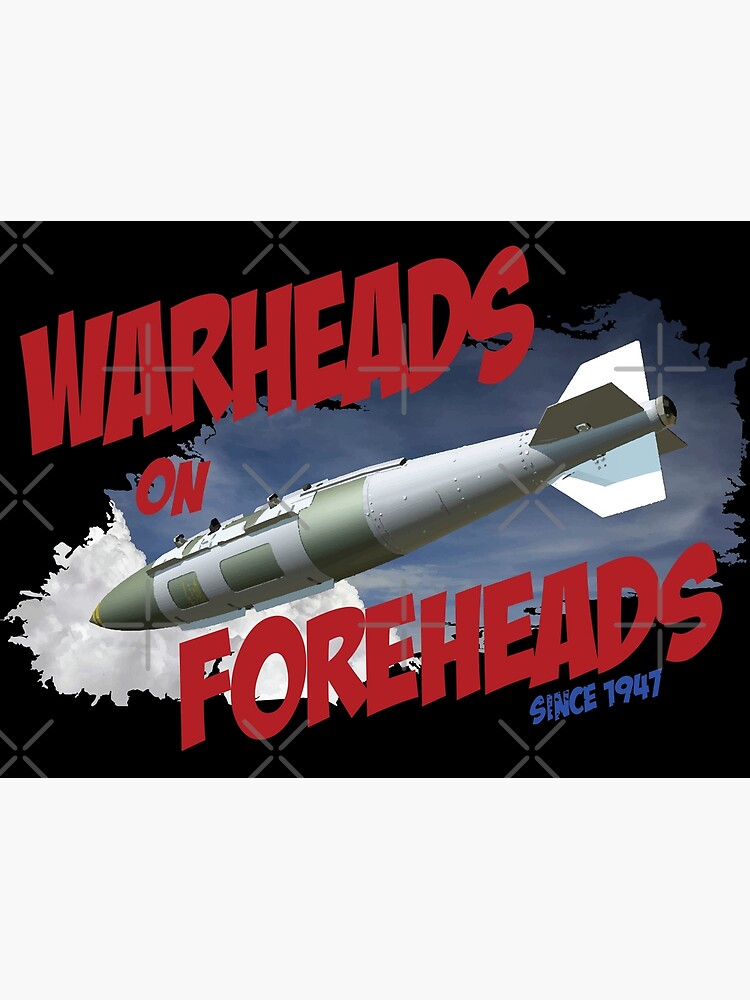This poster features a detailed image evocative of a wartime scene, prominently displaying a missile-like object set against a black background adorned with gray X's and plus signs. The focal point is a warhead, depicted in gray with green accents and a touch of yellow on its tip, seemingly dropping from a bluish sky dotted with clouds. The bold, red uppercase text "WARHEADS ON FOREHEADS" dominates the poster, creating a striking contrast with the blackish backdrop, while below in a smaller purple font, it states "Since 1947." The design, with its gold and white highlights on the missile and intricate decorative elements, suggests a historical or perhaps satirical theme, making it an intriguing and thought-provoking visual piece.